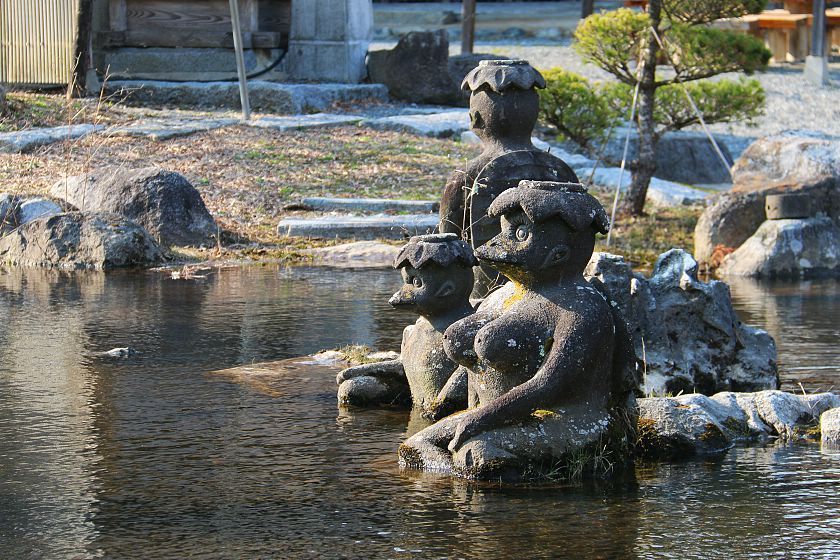This photograph, taken outdoors during the daytime, is a rectangular image measuring approximately six inches wide by four inches high. It features a small brown-colored pond surrounded by tan and white rocks, at the center of which are three statues depicting Japanese Kappa. These humanoid creatures have beaks, leaves for heads, and bowls on top of their heads that typically carry water. All three Kappa statues also have turtle shells on their backs. 

In the forefront, there is a female Kappa sitting down, identifiable by her breasts, who is looking towards the left and holding the hand of a smaller child Kappa, also facing left. The third Kappa stands with its back to the viewer, displaying its turtle shell. 

The upper half of the photograph shows the pond's shore featuring some steps leading upwards, very short cut grass, and a small tree with green leaves surrounded by ropes. The background includes additional rocks and hints of a building, adding context to the outdoor setting. The scene is framed by the tranquil pond and its mythical residents, emphasizing the serene yet mystical ambiance captured in this snapshot.